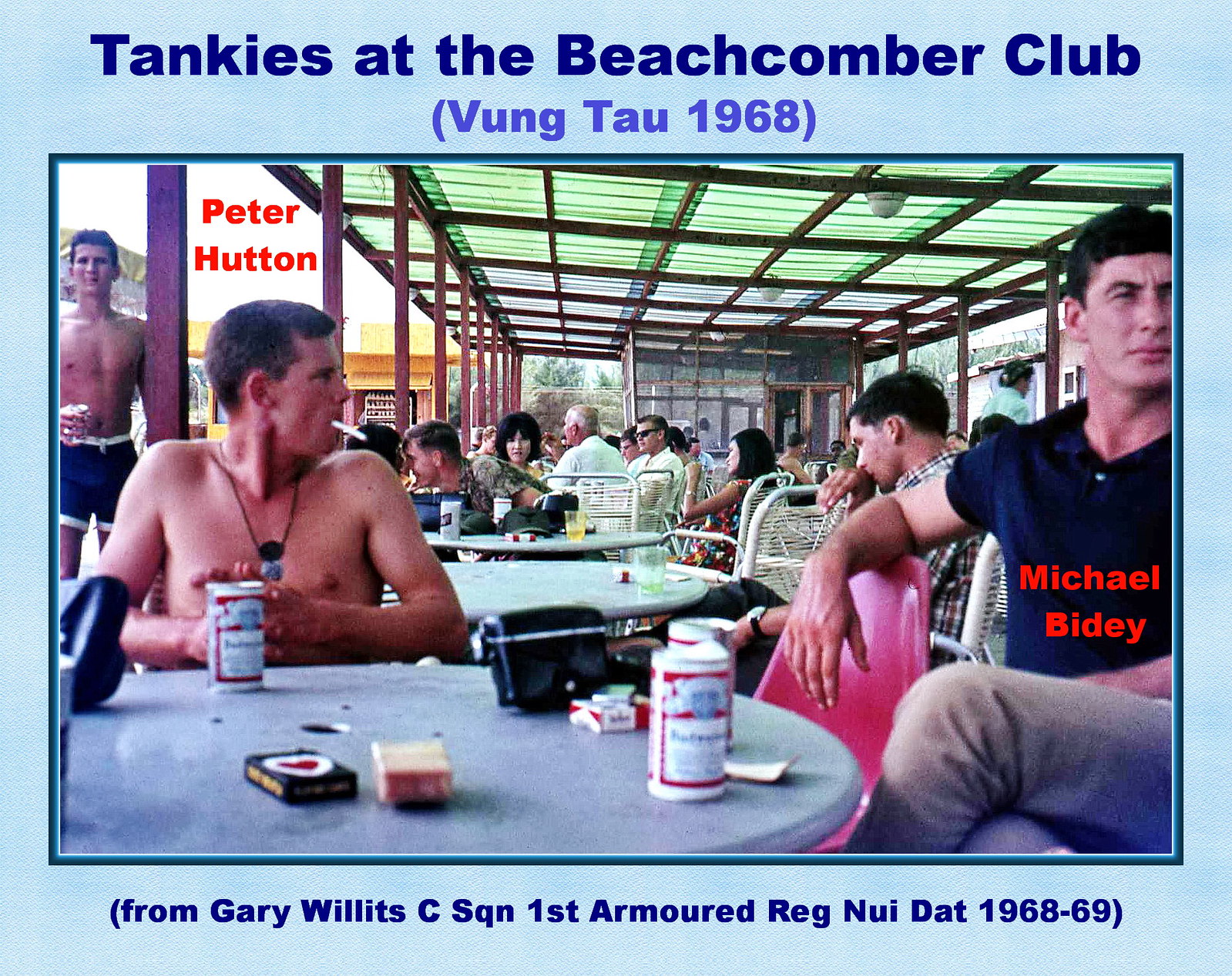The image is a framed photograph with a light blue outer border and a thin dark blue inner border, creating a distinct frame. At the top of the light blue border, blue text reads "Tankies at the Beachcomber Club" with purple text underneath in parentheses noting "Vung Tau 1968." The bottom of the light blue border contains dark blue text in parentheses: "From Gary Willett's C Squadron, First Armored Reg, Nui Dat 1968-69."

The photograph captures a lively open-air eating or picnic area with a clear plastic canopy mounted on a metal brown frame overhead. Several people are seated around tables, including a distinctive pair of men closest to the camera. The man on the right, wearing a blue shirt and jeans, is identified by red text reading "Michael Bidet" over his shirt. The man on the left, shirtless with a black necklace and holding a cigarette, has red text above him that says "Peter Hutton." Both are seen amidst three cans of Budweiser with the iconic white, blue, and red label strewn on the table, along with a pack of Marlboro cigarettes, and what appears to be a pack of playing cards. A purse rests on the table, suggesting a casual and communal atmosphere. More shirtless men in blue shorts and additional individuals, both men and women, populate the background, creating a sense of gathering and camaraderie.